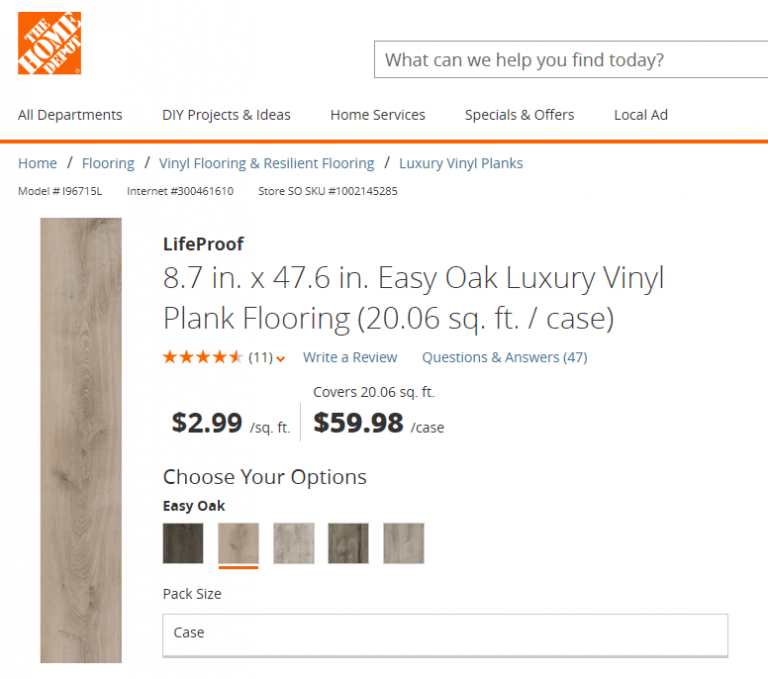This image is a screenshot of the Home Depot website, specifically highlighting a product page. The unmistakable orange Home Depot logo with white diagonal lettering is visible at the top left corner of the page. Adjacent to this logo, at the same horizontal level, is a search bar with the prompt “What can we help you find today?”

Below the main header, the website's navigation options are listed: "All Departments," "Do-It-Yourself Projects and Ideas," "Home Services," "Special Offers," and "Local Ad." The breadcrumb trail below these options reads: "Home," "Flooring," "Vinyl Flooring and Resilient Flooring," "Luxury Vinyl Plank Flooring," indicating the user has navigated to a specific product: Lifeproof Easy Oak Vinyl Plank Flooring.

This highlighted product is described in detail, with its dimensions listed as 8.7 inches by 47.6 inches. The plank is vertical in the displayed image and features a tan and brown oak-like appearance, though made from vinyl. The product name is clearly shown as "Lifeproof Easy Oak Vinyl Plank Flooring." Each case covers an area of 20.06 square feet.

User feedback is provided, with an average rating of four and a half stars from 11 reviews. A “Write a Review” button is also visible, along with a section indicating there are 47 questions and answers available for this product.

Further down, the text reiterates that one case covers 20.06 square feet and provides pricing details: $2.99 per square foot and $59.98 per case. Users are given the option to choose from five different color variations ranging from dark gray to tan, light gray, medium gray, and a whitish-gray option. Below this, there are options for selecting pack size and the number of cases needed.